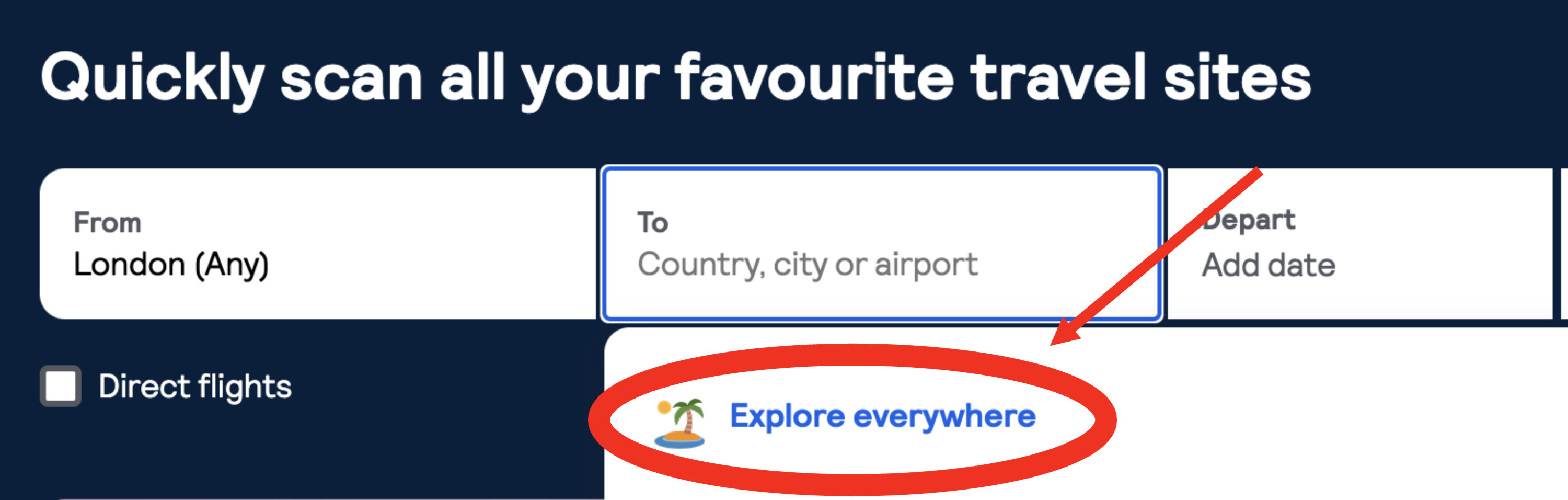The image displays a printout of a webpage, seemingly from a travel site. The design features a dark blue and white color scheme. At the top of the page, the tagline "Quickly scan all your favorite travel sites" is prominently displayed in white text, with "favorite" notably spelled in the British English as "favourite". 

Below the tagline, empty input fields are arranged from left to right: From (London), To (country, city, or airport), and Depart (add date). None of these fields are filled in. Immediately beneath this section, a checkbox for "Direct Flights" is available on the left, while to the right, the phrase "Explore everywhere" is highlighted, next to a photo of a palm tree under the sun. 

A red circle and blue arrow emphasize the words "Explore everywhere", indicating that the user has opted for this travel search feature. Additionally, the arrow points from the "Depart, add date" section, suggesting that this specific travel option has been selected.